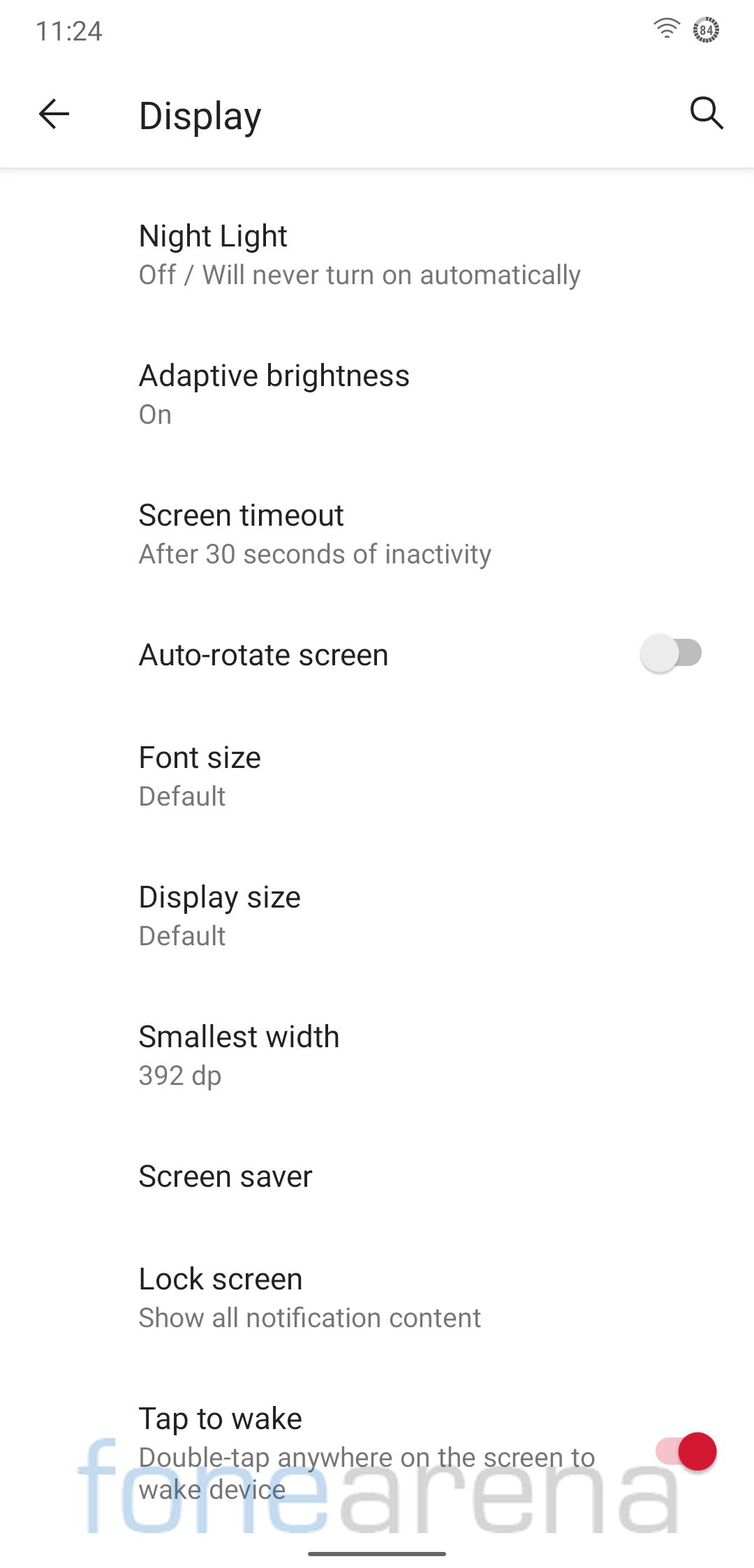In this vertically oriented smartphone screenshot, various settings and notifications from the phone's display settings menu are shown against a white background, which appears to be illuminated by a computer screen. At the top of the screen, the time is displayed as 11:24 on the upper left corner, while the Wi-Fi icon and a circular symbol are visible on the upper right corner. 

On the left side beneath the status bar, there's a 'go-back' arrow followed by the word "Display," with a magnifying glass situated on the upper right. Below this section, a dividing line is present.

The following settings are listed with their respective statuses:

- **Night Light** (in black) with **Off / Will never turn on automatically** (in gray) underneath.
- **Adaptive Brightness** (in black) with **On** (in gray) underneath.
- **Screen Timeout** (in black) with **After 30 seconds of inactivity** (in gray) underneath.
- **Auto-Rotate Screen** (in black) with a toggle indicating it is currently off.
- **Font Size** (in black) with **Default** (in gray) underneath.
- **Display Size** (in black) with **Default** (in gray) underneath.
- **Smallest Width** (in black) with **392 dp** (in gray) underneath.
- **Screensaver** (in black).
- **Lock Screen** (in black) with **Show all notification content** (in gray) underneath.
- **Tap to Wake** (in black) with **Double-tap anywhere on the screen to wake device** (in gray) and a red toggle button indicating it is on.

At the very bottom of the image, the text "Phone Arena" can be seen.